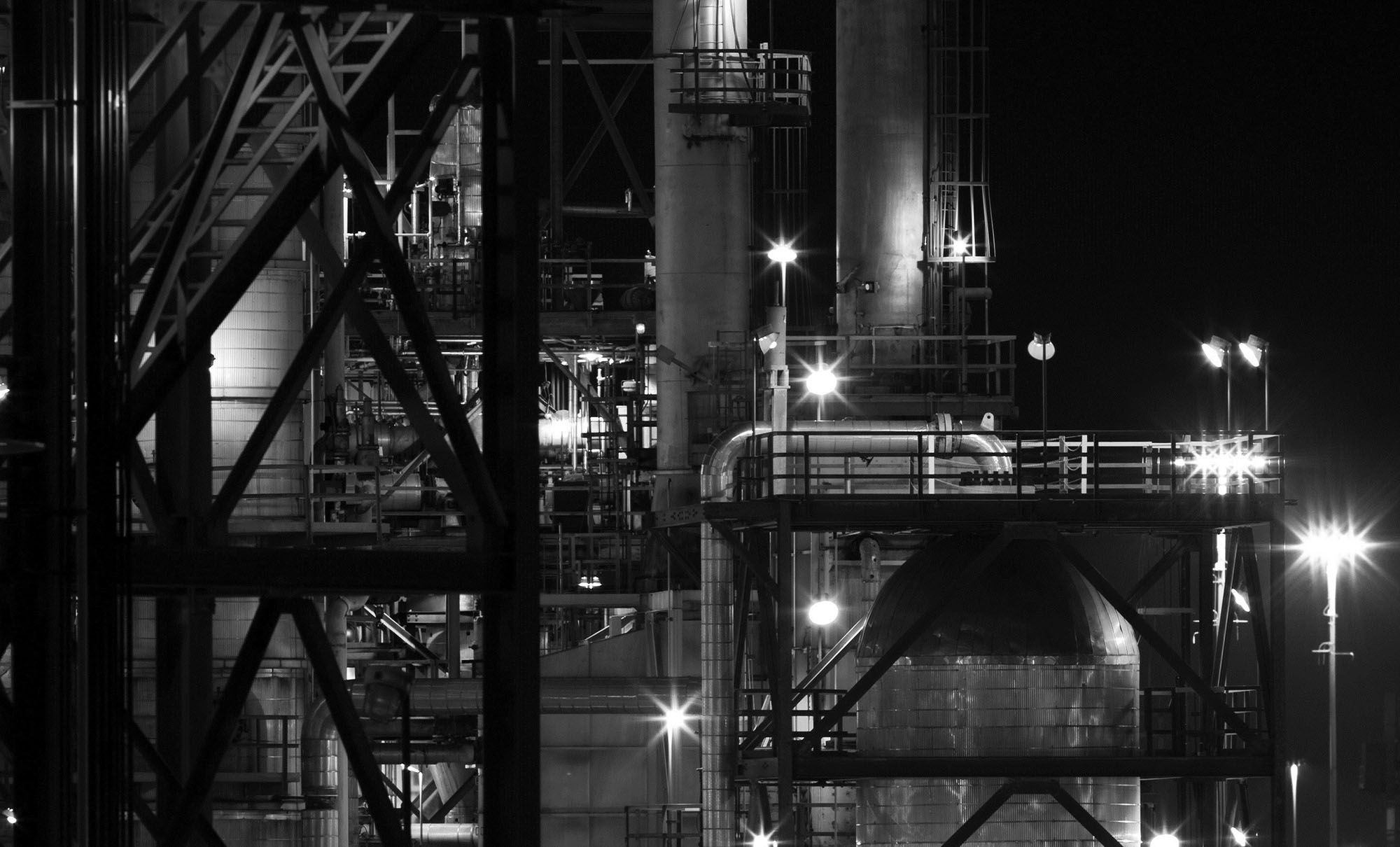A detailed nighttime black and white photograph capturing an industrial plant or factory. The image is dominated by tall metal towers and cylinders, which likely serve as part of a power generation facility. In the foreground, there are intricate arrangements of scaffolding, steep metal steps, and ladders crisscrossing the scene. Bright lights and spotlights illuminate the facility, casting stark, glowing auras against the dark backdrop. Metal pipes, possibly transporting gas or liquid, weave through the setup, connecting different sections of the plant. The photograph's center showcases two prominent metal towers, with an additional metal cylinder and pipe system to the lower right. The overall ambiance of the image emphasizes the intense industrial activity and the meticulous structural design typical of such environments.